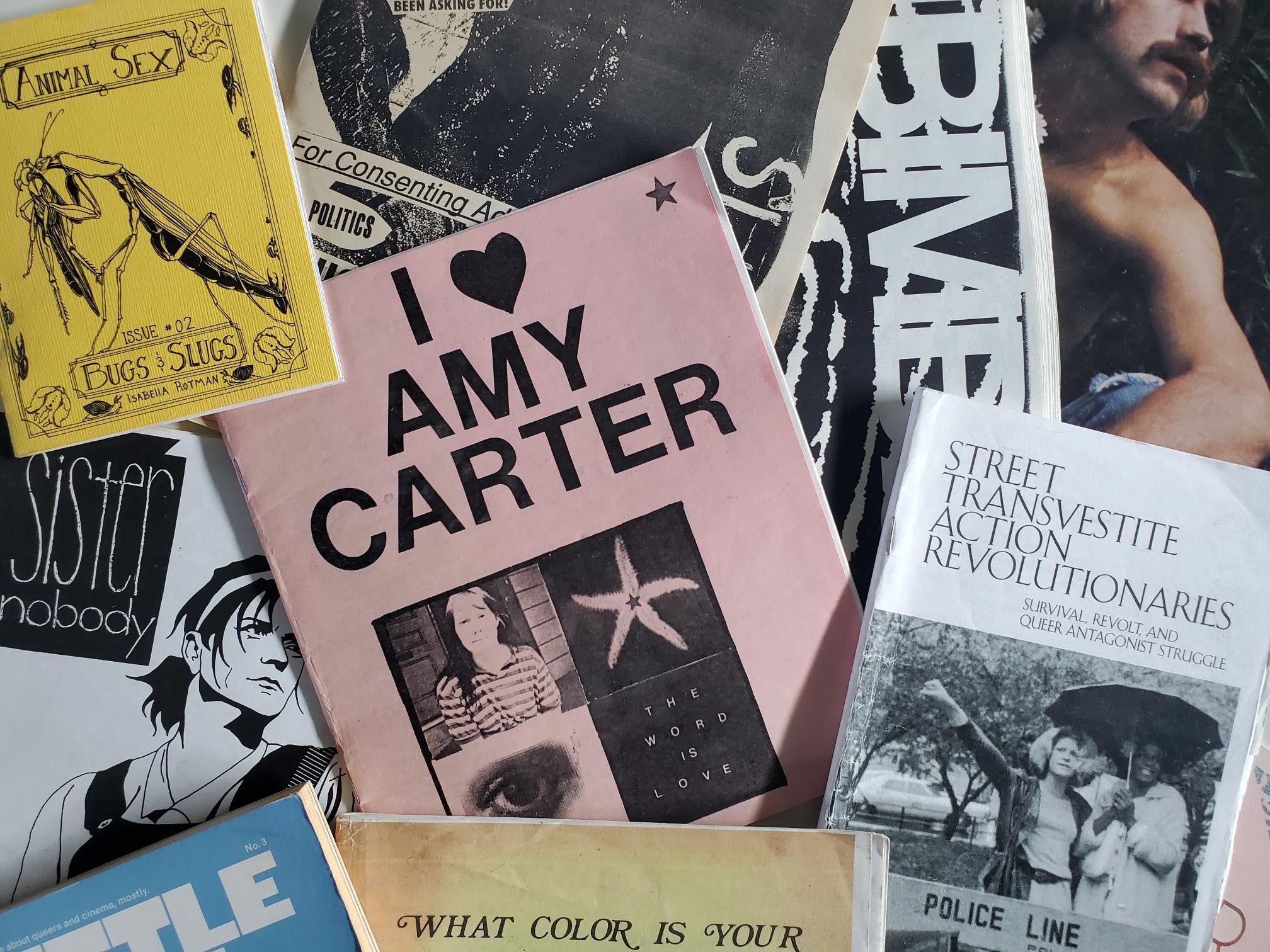This image features a haphazardly arranged collection of small zines and booklets stacked together. Prominently, a pink zine titled "I Heart Amy Carter" sits in the center, adorned with a star sticker in the upper right and images of a woman in a striped shirt, a sea star, an eyeball, and text saying, "the word is love." To the upper left, a yellow zine titled "Animal Sex" with the subtitle "Bugs and Slugs" is labeled as issue number 02 and shows a praying mantis, likely engaging in predatory behavior with another mantis. The author's name appears but is too small to decipher clearly. Partially covered by the other zines, one titled "Sister Nobody" features a confident-looking woman drawn on the cover. In the lower right corner, another zine, "Street Transvestite Action Revolutionaries," showcases two women, one with an umbrella and the other raising a fist, alongside a police line, with the subtitle "Survival Revolt and Queer Antagonist Struggle." Additionally, there are several more obscured zines in the background, one which reads "For Consenting and Politics," another showing "B-I-M-A-B" partially, and one featuring a shirtless man. All these zines create a colorful and eclectic visual display.